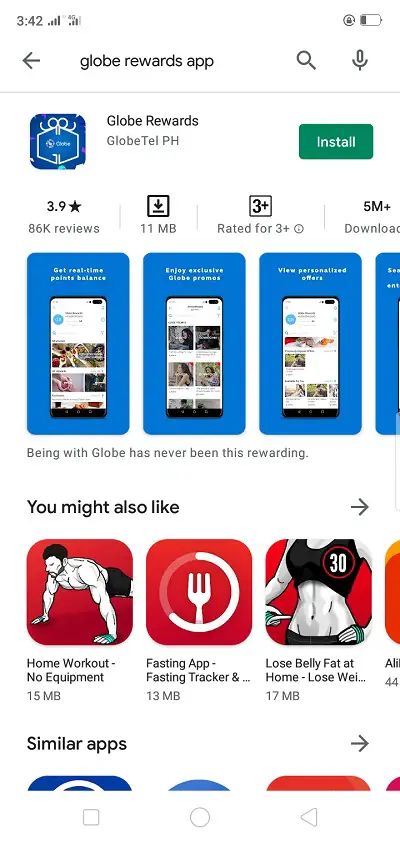A clear, detailed mobile app interface showcasing the "Globe Rewards" app on a white background. The app features a rating of 3.9 stars based on 86,000 reviews, and a size of 11 MB, suitable for users aged 3 and above. It boasts over 5 million downloads. Prominent app features include a green "Install" button and icons for search, microphone, and navigation on the screen. 

The main display highlights the app's slogan "Being with Globe has never been this rewarding." accompanied by four illustrative screenshots with a vibrant blue background. Under the "You Might Also Like" section, suggestions for other apps include "Home Workout - No Equipment" (15 MB), "Fasting App - Fasting Tracker" (13 MB), "Lose Belly Fat at Home" (17 MB), and various weight loss and fitness apps, indicated with a "..." for truncation.

At the lower portion of the screen, a navigation bar features additional options and a right arrow for exploring similar apps. This portion shows four app suggestions in a grid format. The bottom navigation bar includes a square, a circle, and a triangle within a left arrow configuration for further user engagement.